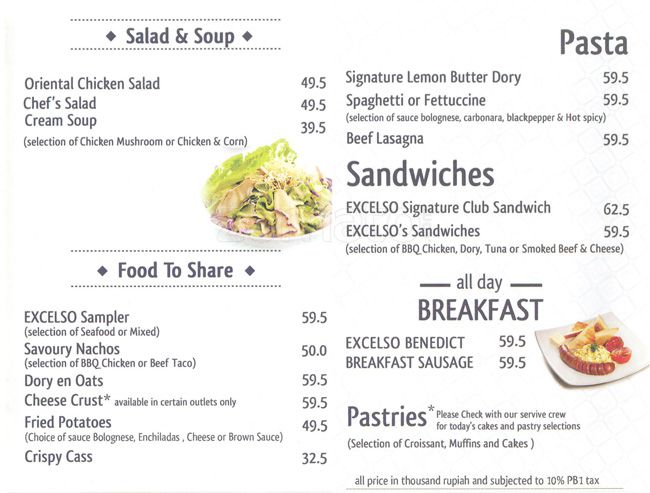This is a horizontal rectangular menu image with a predominantly white background and faint borders on the left side and bottom. A subtle diamond pattern adorns the right side of the page. On the left, two main categories are highlighted with bars and diamonds on the top and bottom: "Salad and Soup" and "Food to Share." 

Under "Salad and Soup," dishes listed include:
- Oriental Chicken Salad, 49.5
- Chef's Salad, 49.5
- Cream Soup (Chicken Mushroom or Chicken and Corn), 39.5

Depicted is a plate of chicken salad. "Food to Share" features items such as:
- Excelso Sampler (seafood or mixed), 59.5
- Savory Nachos (barbecued chicken or beef taco), 50.0
- Dory and Oats, 59.5
- Cheese Crust (available in certain outlets only), 59.5
- Fried Potatoes (choice of sauce: bolognese, enchiladas, cheese or brown sauce), Crispy Cass, 49.5
- Crispy Cass, 32.5

The right side of the menu presents sections such as "Pasta," "Sandwiches," "All Day Breakfast," and "Pastries." 

Under "Pasta," selections include:
- Signature Lemon Butter Dory, 59.5
- Spaghetti or Fettuccine (sauce choices: bolognese, carbonara, black pepper, hot and spicy), 59.5
- Beef Lasagna, 59.5

Under "Sandwiches," items listed are:
- Excelso Signature Club Sandwich, 62.5
- Excelso Sandwiches (barbecued chicken, dory, tuna, or smoked beef and cheese), 59.5

The "All Day Breakfast" section features:
- Excelso Benedict, 59.5
- Breakfast Sausage, 59.5

There's a plate with what appears to be sausages. The "Pastries" section notes an asterisk, advising patrons to check with the service crew for the daily selection of croissants, muffins, and cakes.

At the bottom right corner, a note states that all prices are in 1,000 rupiah and subject to a 10% PB1 tax.